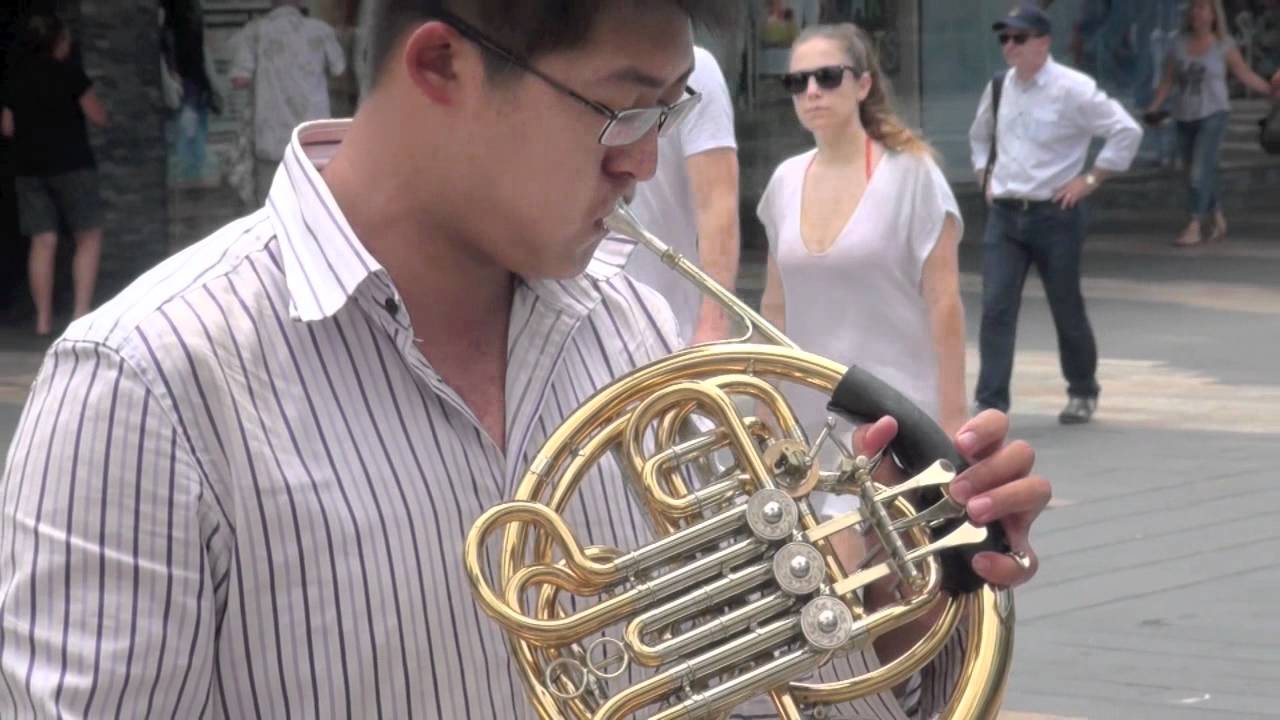In a bustling city square, an Asian man with black hair and glasses is captured mid-performance, playing a French horn. He wears a white collared shirt with vertical black, blue, and thin gray stripes. His French horn is gold and silver, featuring a black grip. With his third finger pressing down on one of the horn's three valves, he blows into the instrument, fully immersed in his music. Surrounding him, a variety of people are seen walking, adding to the lively atmosphere of the public space. Notably, a white woman in sunglasses and a white blouse, revealing a bikini underneath, glances at the performer as she strolls by. Close behind her, a white man in a collared shirt, jeans, a satchel, and a bob cap, also sporting sunglasses, walks with his hands on his hips. The background, a cement promenade, is filled with other passersby, contributing to the dynamic urban scene.